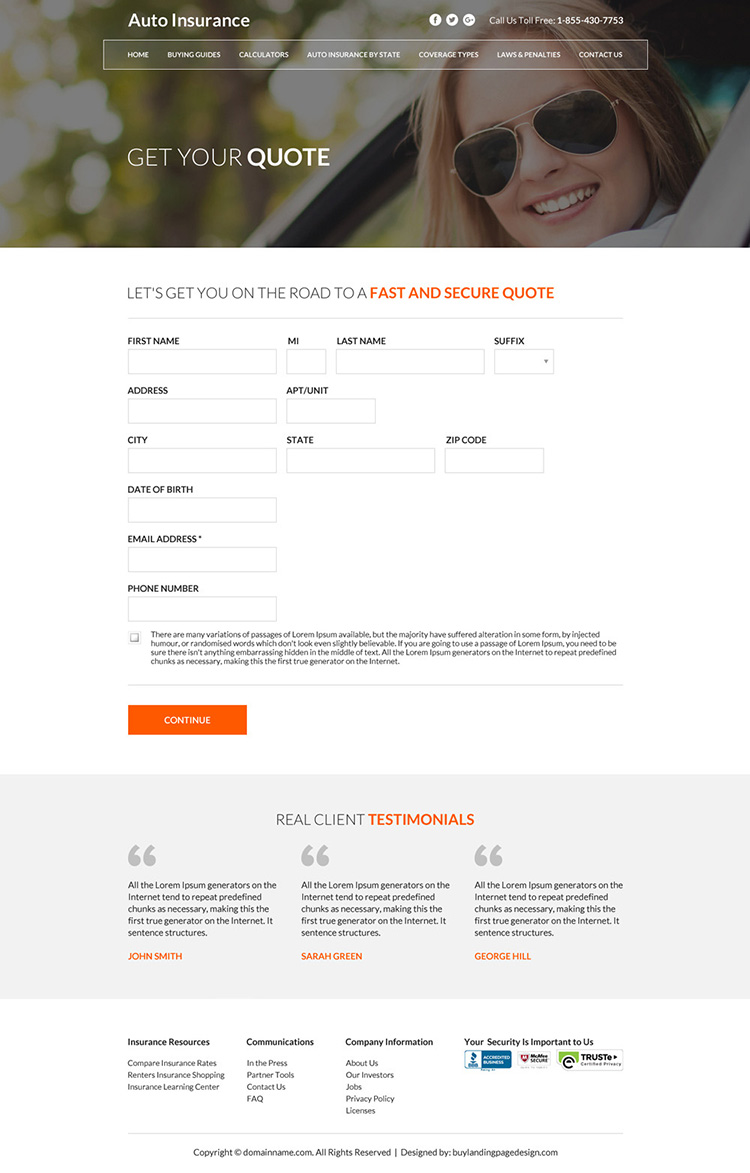This image appears to be a screenshot of a computer screen displaying a webpage for an auto insurance company. At the top of the page is a banner featuring a partially blurred image to the left, where green and white circles are vaguely visible. On the right side of the banner, there is a picture of a woman with long blonde hair, wearing sunglasses, looking out of a car window towards the viewer. In the upper left corner of the banner, the text "Auto Insurance" is visible, with a phone number positioned to the right of it.

Below the banner, a horizontal menu bar spans the width of the screen. At the bottom of the banner, a call-to-action button reads "Get Your Quote." Beneath this, there is a white section with the header "Let's Get You On The Road to a Fast and Secure Quote," with "Fast and Secure Quote" highlighted in orange. This section contains several input boxes prompting for detailed personal information including first name, middle initial, last name, suffix, address, apartment number, city, state, zip code, date of birth, email address, and phone number. Completing this form appears to lead to an orange "Continue" button.

Further down the page, there's a gray rectangle labeled "Real Client Testimonials," under which three paragraphs of testimonials are arranged horizontally. At the very bottom of the screen, a white footer is divided into three sections: "Insurance Resources," "Communications," and "Company Information." An additional note reassures users with the statement, "Your security is important to us."